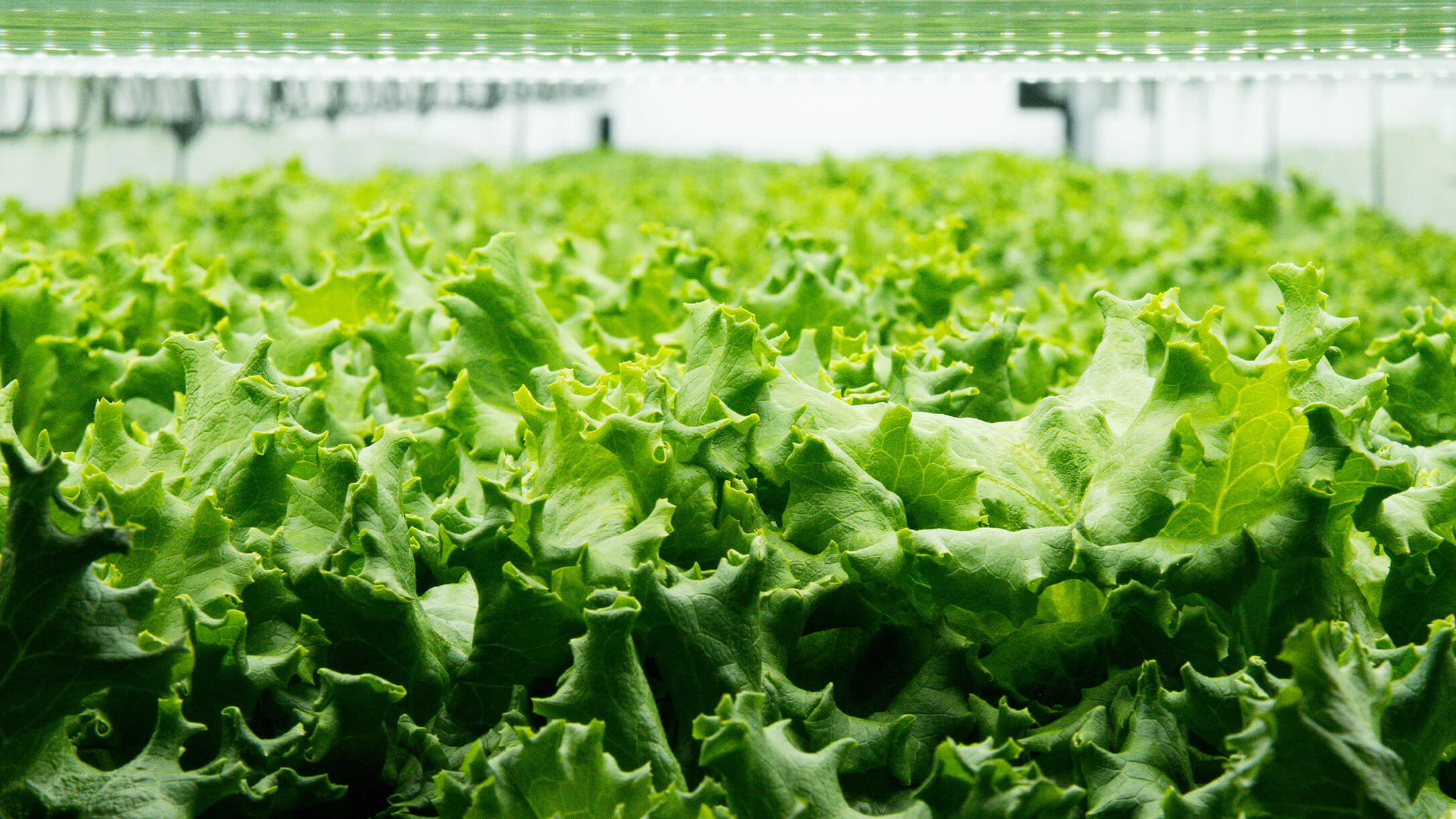The photograph depicts a vibrant, close-up view of a greenhouse brimming with green lettuce leaves. The prominently featured leaves are large and intricately curled or twisted, revealing a yellowish hue along their edges where the light hits. The image offers a clear view of the lush, green lettuce at the forefront, while the background progressively blurs out, accentuating the dense foliage. Surrounding the leafy greens, a white plastic fencing or wall can be seen in the distance, suggesting an indoor farming environment. The scene is brightly lit, with light emanating from a low, plasticky ceiling above, casting a natural illumination that highlights the healthy, verdant leaves. The overall setting of the greenhouse imparts a sense of an organized, well-maintained farm dedicated to cultivating rows of lettuce in optimal conditions.